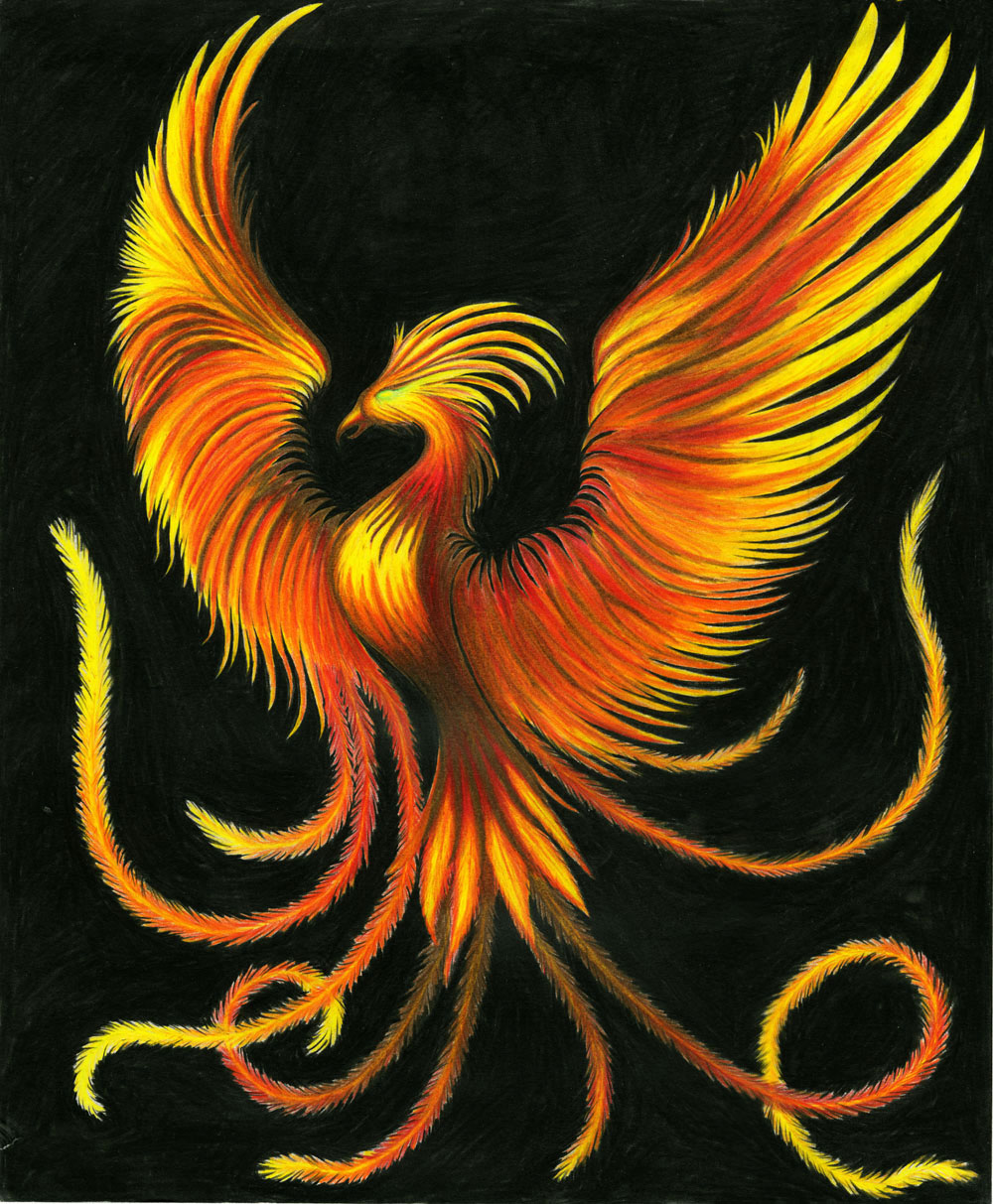This is a detailed artwork depicting a mythical phoenix set against a pure black background. The bird, predominantly yellow and orange with accents of red and gold, faces the left side of the image. Its wings are dramatically outstretched and arched upward, giving a powerful and triumphant appearance. The feathers are wispy and flame-like, creating the illusion of fire. The phoenix's sharp beak, painted in a striking orange, complements its intense green eye. The bird's chest is proudly puffed out, adding to its ferocious and majestic demeanor. Instead of legs, the creature has multiple, snake-like appendages that curl and wind around, extending in various directions. These appendages blend from fiery yellows at their tips to deeper oranges and reds near the body, enhancing the bird's vibrant and otherworldly presence. The entire composition is slightly taller than it is wide, emphasizing the phoenix's verticality and grandeur.